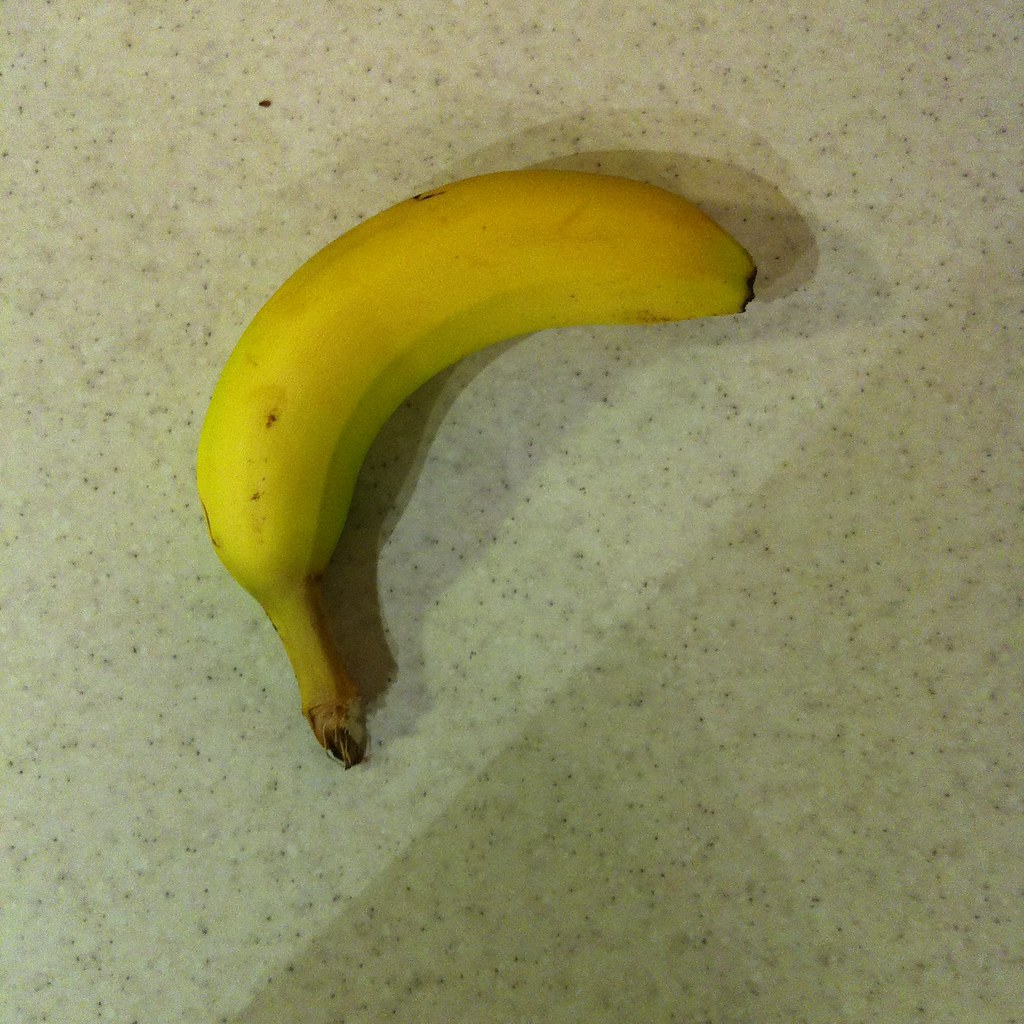A square, medium-quality portrait-style photograph features a yellow banana with light brown speckling. The banana, which appears to be slightly unripe with a greenish tint on the inside, is positioned upside down. The stem of the banana is facing towards the middle bottom of the image, while the curved body of the banana lays parallel to the bottom edge, pointing to the right. The banana casts a subtle shadow on a peppered granite countertop. The countertop's base color is a blend of greyish light khaki, interspersed with lighter black speckles, adding texture to the background.